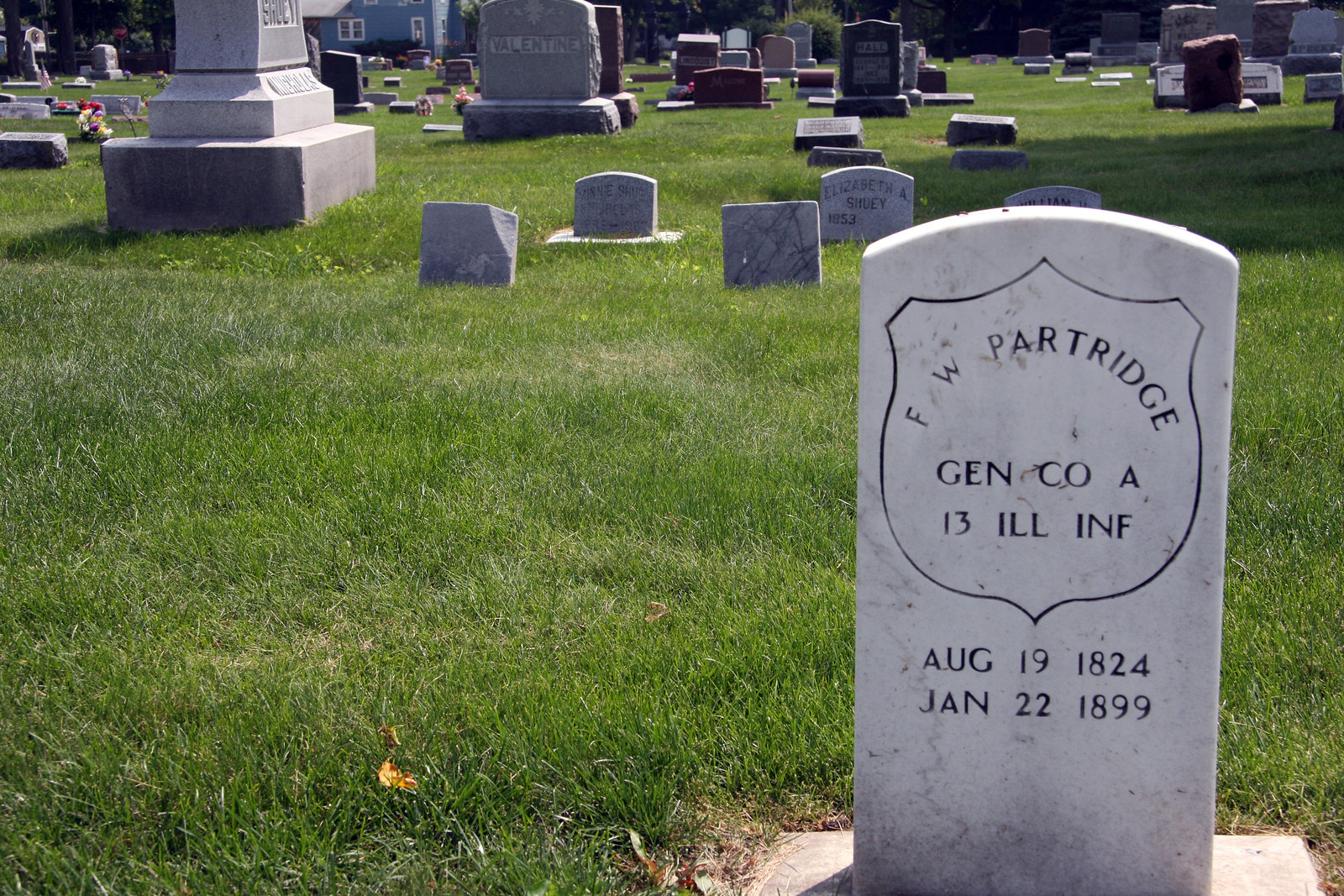This vibrant, well-kept cemetery is filled with numerous gravestones, set against lush, bright green grass. The focal point of the image is the prominent white marble gravestone situated in the foreground on the right side. The gravestone features a shield shape with the inscription "F.W. Partridge, Gen. Co. A, 13 I.L.L. I.N.F." and dates "August 19, 1824 - January 22, 1899." The headstone's detailed lettering and design stand out against the backdrop of various other tombstones scattered throughout the cemetery, some larger and some smaller, some upright and some laid flat. The sun casts shadows across the scene, highlighting the contrast between the gravestones and the greenery. In the upper left corner of the image, there's a blue house with white trim, adding a touch of color to the background. Near the house, a few flowers and bushes complete this serene resting place.